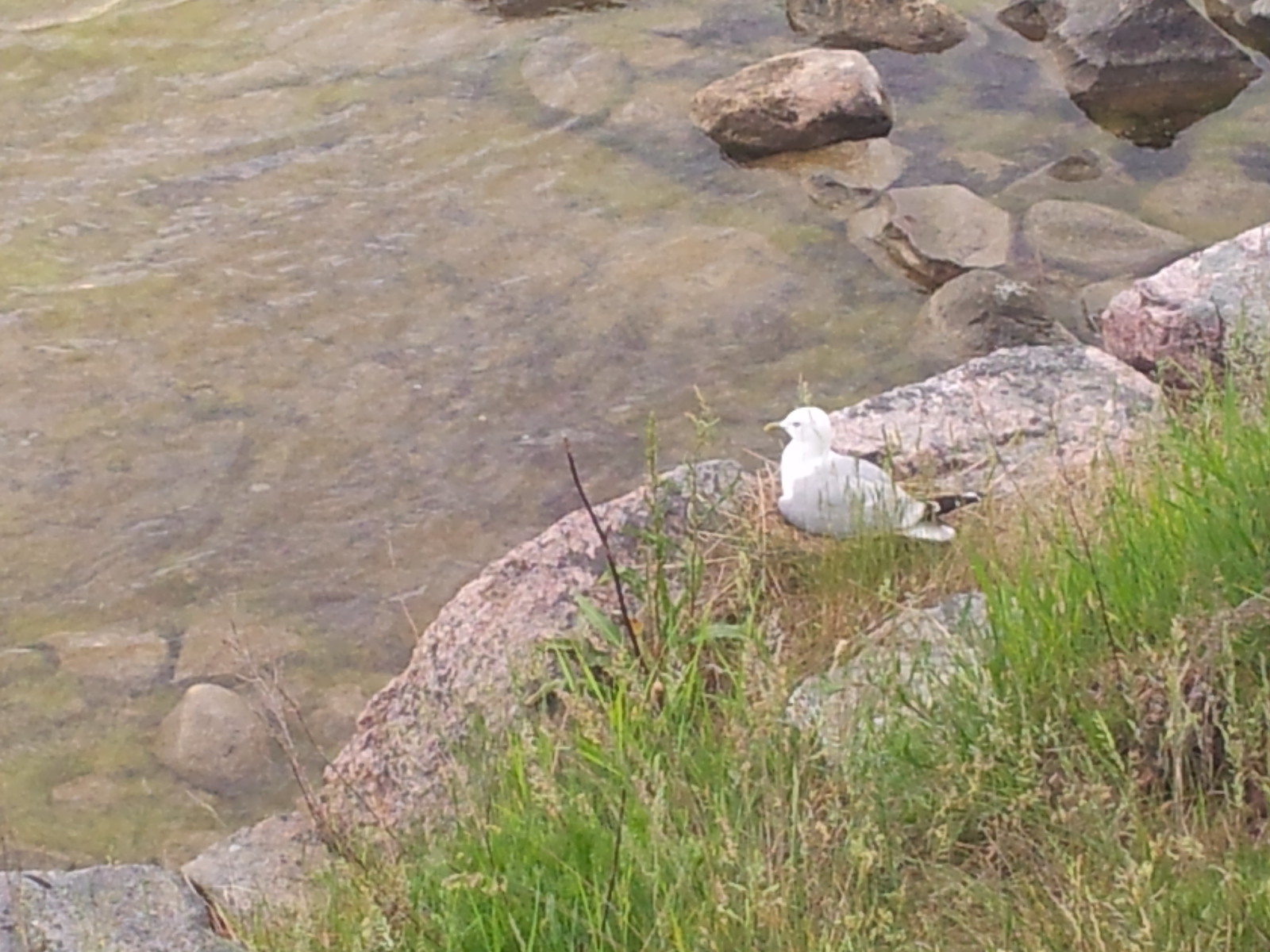In this detailed photograph, there's a serene creek occupying the upper left portion, where shallow, slightly muddy water reveals rocks beneath the surface. The water extends to the upper right, interspersed with partially submerged and exposed rocks. A notable feature in the middle of the image is a man-made beige and gray brick barrier. Perched on this barrier is a seagull, identifiable by its white body, gray wings, black tail, and yellow hooked beak, seemingly gazing at the water. In the bottom right portion behind the seagull, there's a patch of tall, unkempt green and brown grass, which appears somewhat neglected. Among the grass, a single rock is partially buried. The overall calm of the scene is subtly disrupted by ripples in the water, suggesting a gentle current.